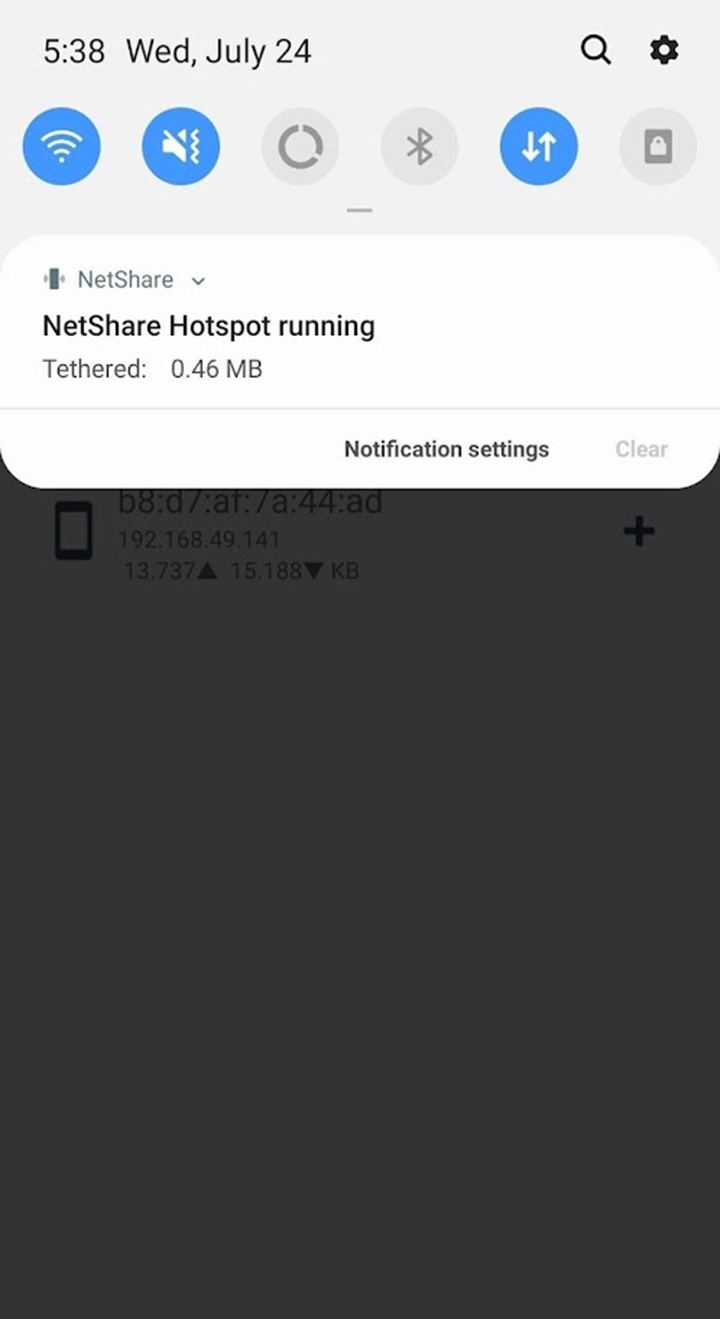The description provided needs better organization and detail. Here's an enhanced and organized version of the caption:

---

The image is a screenshot of a mobile app displayed on a vertically oriented smartphone screen, divided into several distinct sections.

At the very top, there is a gray bar spanning the width of the screen. On the left side of this bar, the text reads "538, WD, July 24." The right side contains two icons: a magnifying glass representing the search function and a daisy wheel symbolizing the settings.

Below this gray bar, there is a row of circular buttons, some blue and some gray. From left to right, the buttons are:
1. A blue Wi-Fi icon.
2. A blue icon depicting a crossed-out volume symbol.
3. A gray Bluetooth icon.
4. An unidentified gray icon.
5. A blue icon with an up and down arrow, likely indicating scroll functionality.
6. A final gray icon that resembles either a lock or a bag.

Beneath the row of buttons, there is a white box containing more detailed information. This box reads "NetShare" at the top and "NetShare hotspot running" below it. Further down within the same box, it states "Tether 0.46 MB" on the left side, while on the right side, there are options for "Notification settings" and a clear button, likely to dismiss notifications.

The lower portion of the screenshot appears shaded or blacked out, obscuring any additional information that might be present.

---

This structured format provides clarity and context for each section of the screenshot, making it easier to understand.